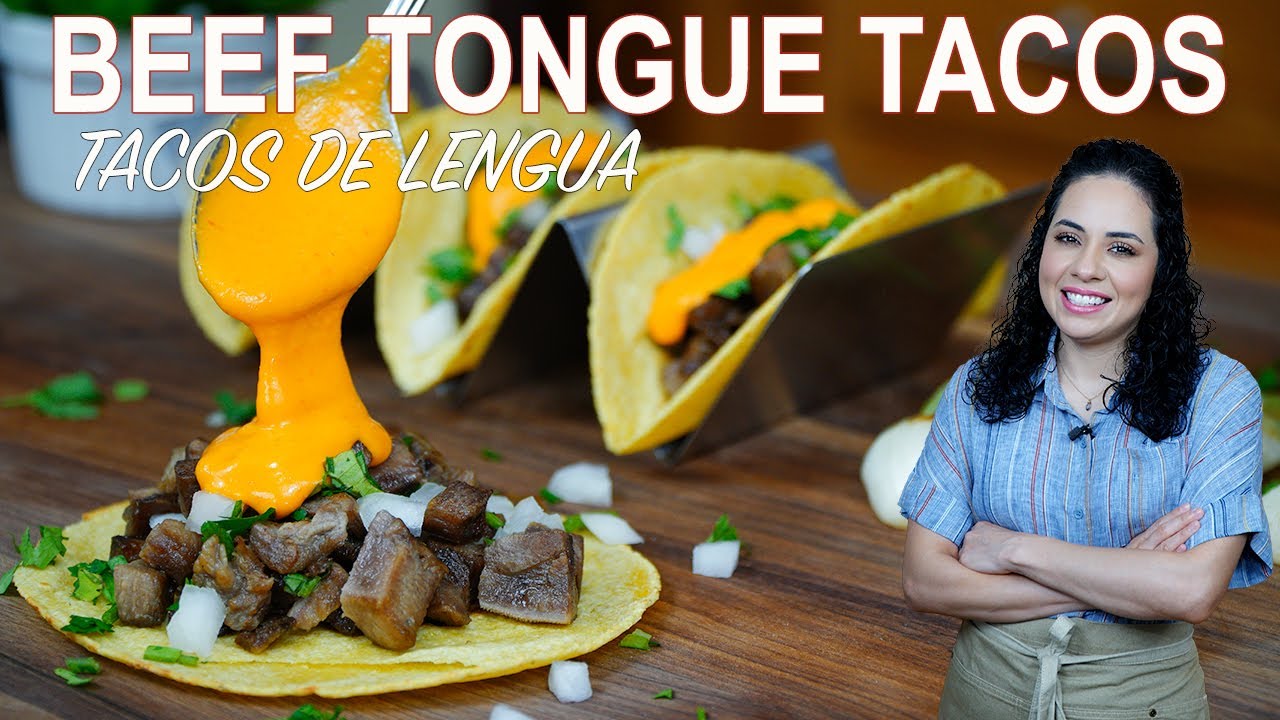In this advertisement for tacos, the main highlight is the tantalizing presentation of Beef Tongue Tacos, accentuated by the headline "Beef Tongue Tacos" in large white letters across the top, and "Tacos de Lengua" underneath in smaller white text. Dominating the left side of the image, a close-up showcases a taco with beef, white onions, lettuce, and a spoon pouring cheese over the meat. Behind this foreground taco, three tacos are neatly arranged in a V-shaped metal holder, topped with beef, green shredded parsley, and queso cheese. A white ramekin filled with green herbs is also visible, enhancing the fresh appeal of the dish. On the right side of the image stands a woman with long black hair, smiling warmly at the camera. She is wearing a blue button-up shirt with red and blue stripes and a brown skirt. Her arms are crossed above her waist, and she is positioned in front of a brown table that stretches across the background, adding depth to the overall composition. The blend of culinary allure and welcoming personal touch creates an inviting scene that draws attention to the delicious Beef Tongue Tacos being advertised.